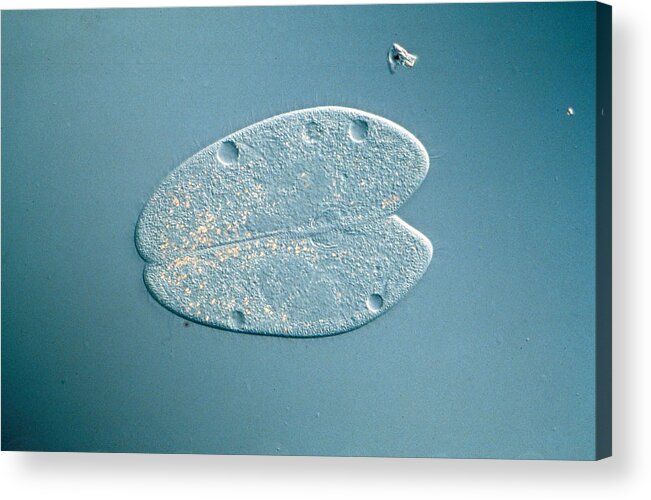The image is a painting with a light blue to seafoam green background, slightly darker in the upper right and lower left corners. At the focal point of the painting is a heart-like structure, resembling a pair of cells that seems to be in the process of splitting or fusing. This central form consists of two oval shapes with rough, textured surfaces, which are mirrored top and bottom, and each featuring two distinct circles or holes at the top, giving a sense of transparency. The entire form exudes a feeling of organic, almost microscopic life. Above this main figure, towards the upper right, there is a white triangular shape and a small circular dot about a quarter way down from the top right corner, reminiscent of dust or an intentional mark by the artist. The painting is stretched over a rectangular frame with no indication of its size due to the lack of surrounding context.